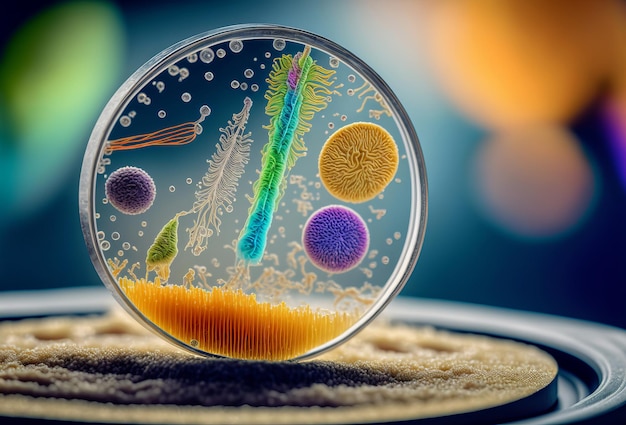This image is a highly detailed, close-up portrayal of a petri dish filled with an array of colorful, germ-like forms, resembling a combination of real and digitally rendered microorganisms. The circular petri dish is arranged diagonally on a textured base that appears to be wood-like, all set against a blurred background featuring faded splashes of blue, green, and orange.

Inside the petri dish, a multitude of intricate forms coexist. The foreground features clear bubbles and various germs or viruses: a jellyfish-shaped orange one, a purple popcorn-shaped one, a light green leaf-shaped form, and orange frillies at the bottom. Above the frillies is a larger, popcorn-like purple germ, adjacent to an orange, sponge-like structure. Another standout is a vibrant, oblong germ showcasing a gradient from cyan to bright green, and back to cyan, with elements of purple and orange. Greenish-yellow frillies adorn its sides. Flanking this multicolored entity are a white, squiggly germ and another purple one. The base texture and blurred background give an impression of depth and subtle realism, elevating the captivating, almost surreal depiction of what might be seen under a high-powered microscope.